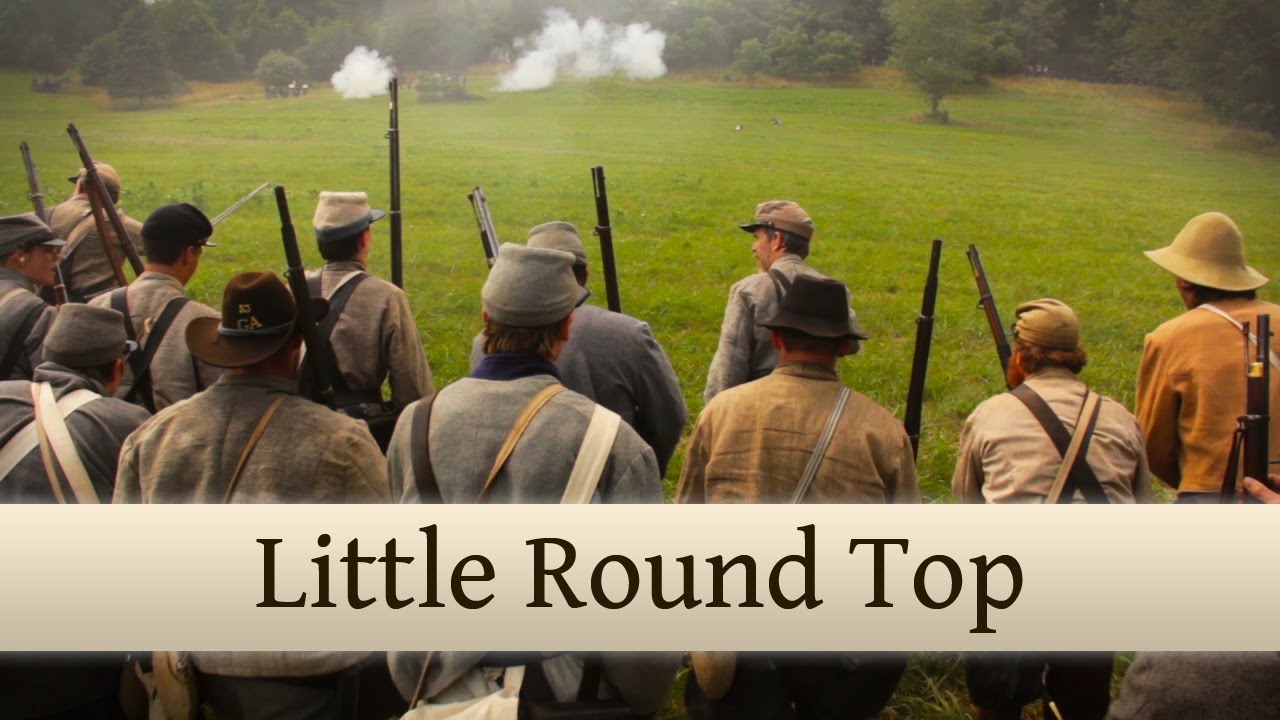This is a color photograph of a Civil War reenactment depicting a group of approximately ten Confederate soldiers standing in the foreground, all with their backs to the camera. They are distinguishable by their gray and makeshift uniforms, complete with suspenders, carrying straps, various caps, and old Civil War-era rifles that shoot musket balls. One soldier on the left is slightly turned, showing his profile. The soldiers are standing in a large, open, green field, gazing at a scene enveloped in smoke from gunfire and cannons. In the far background, more soldiers can be seen, seemingly waiting and poised for an impending clash. The backdrop includes a number of tall green trees. A banner near the bottom of the image reads "Little Round Top," indicating the historical significance of the depicted scene. There are no animals, buildings, or additional text visible in the photograph.